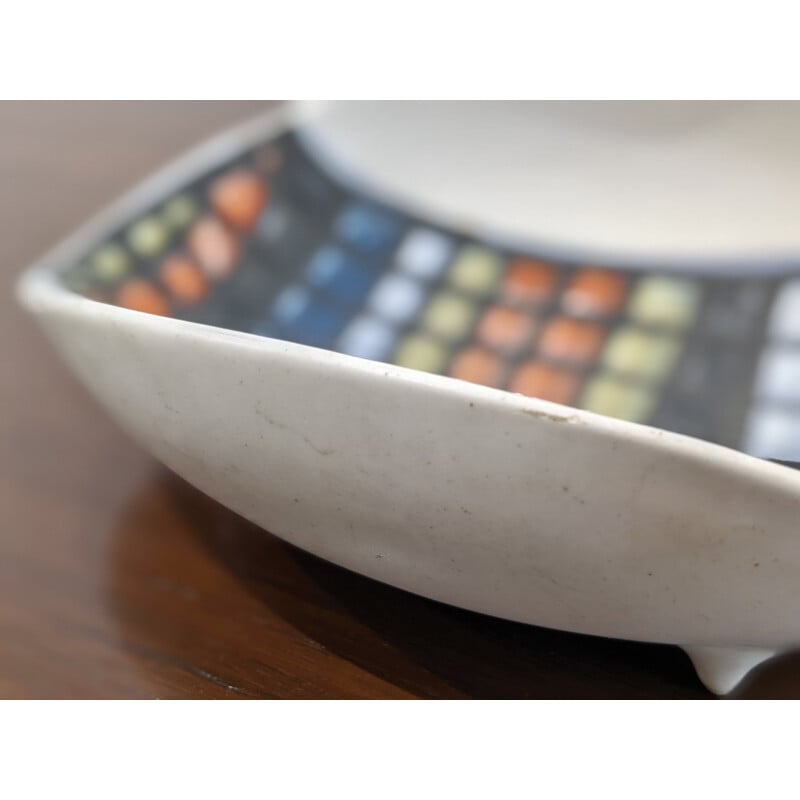The image showcases a close-up of a rustic, white ceramic bowl with three visible legs. The bowl, positioned on a dark brown wood-grain table that is slightly blurred, emanates a warm and antique aesthetic, enhanced by a small chip at the rim and curved edges. Though the outer portion facing the camera is sharp and detailed, the inner part of the bowl is blurred, revealing a captivating mosaic of colorful dots and squares. These colors, including hues of orange, yellow, black, blue, and white, form a vibrant pattern that spans the inner surface, though the details are somewhat obscured by the focus. The intricate design suggests a decorative purpose more than a functional one, making it an alluring piece that balances both artistic allure and vintage charm.